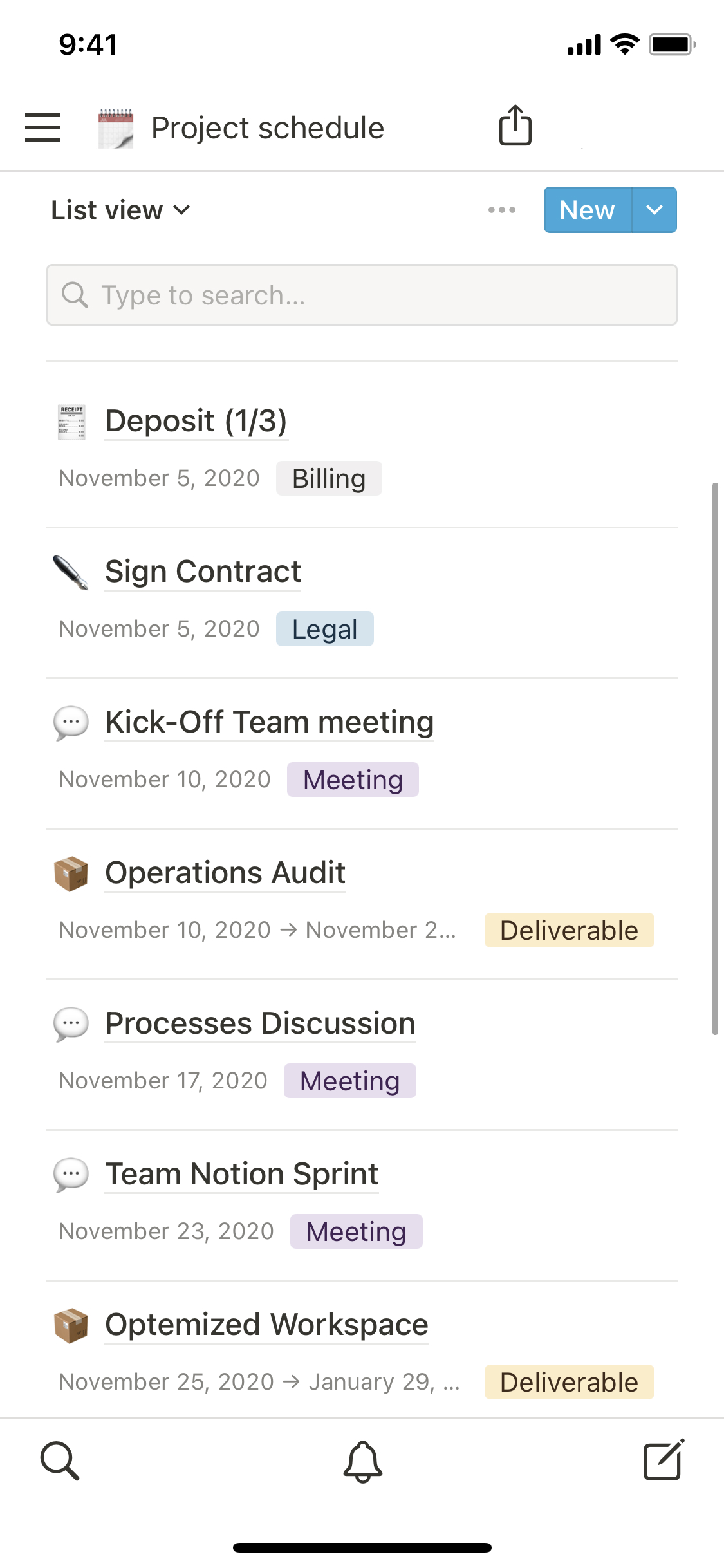This detailed screenshot captures a project schedule in list view, prominently featuring key dates and tasks. In the top right corner, the time is displayed as "9:41." Below, the project schedule is outlined with a series of labels and milestones. 

- "New Deposit" appears first, marked as "1 out of 3," with an associated date of November 5th, 2020.
- Following this, "Billing and Signed Contract" is also dated November 5th, 2020, under the "Legal" category.
- The "Kickoff Team Meeting" is scheduled for November 10th, 2020, classified under "Meeting."
- An "Operations Audit" is listed on the same date, November 10th, 2020.
- On November 2nd, a "Deliverable Process Discussion" is noted.
- A "Team Motion Sprint" meeting is set for November 17th, 2020.
- "Optimized Workspace" is the final meeting listed, occurring on November 23rd, 2020.
- A significant deliverable is projected for January 29th, 2021.

At the top of the screenshot, there are options like "Search," "Notifications," and "Copy." The interface has a black line at the bottom indicating a scroll bar on the right, and the toolbar at the top features a blue background with selections such as "Next" and "New."

The meticulous layout and color-coded organizational cues make this an effective tool for tracking project progress and key activities.